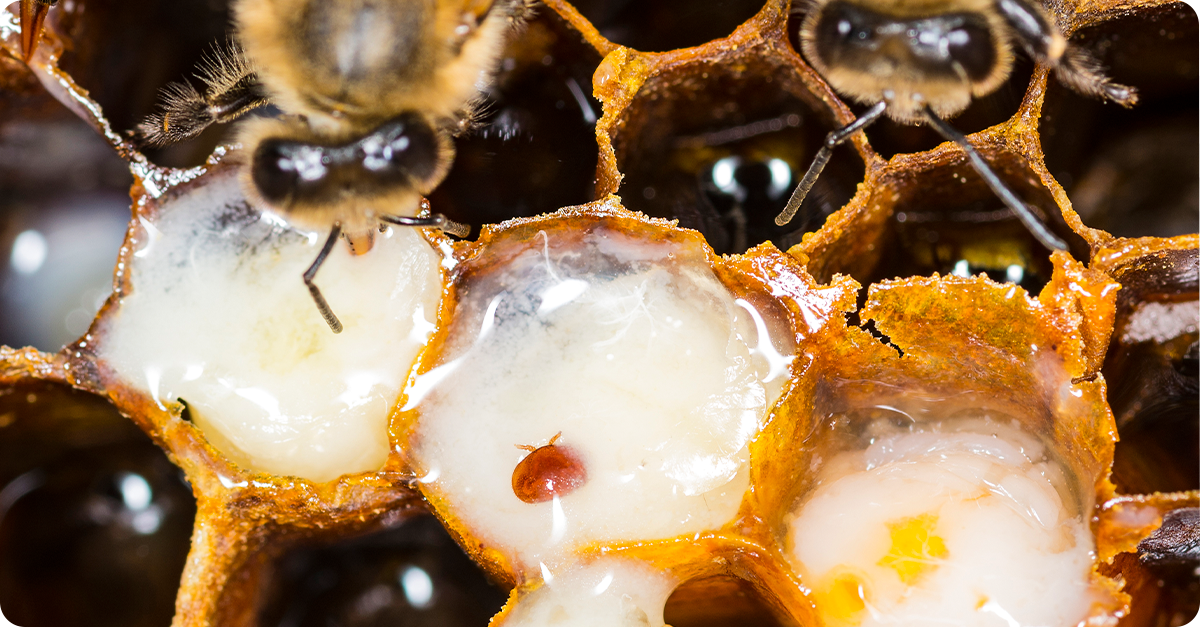This image provides a very detailed close-up of a piece of beehive honeycomb structure. Within the honeycomb, we see an adult bee, yellow and fuzzy, tending to the brood cells. These hexagonal, comb-like structures house numerous immature bees. Several of the cells contain translucent white, gelatinous substances, revealing orange and yellow details of larvae developing within. Some larvae are still growing, while others are in the process of hatching. Amidst this, other bees can be seen walking around, tending to the needs of the colony. The honeycomb itself has a yellow-brown color, adding to the vivid depiction of bustling activity within this miniature world.